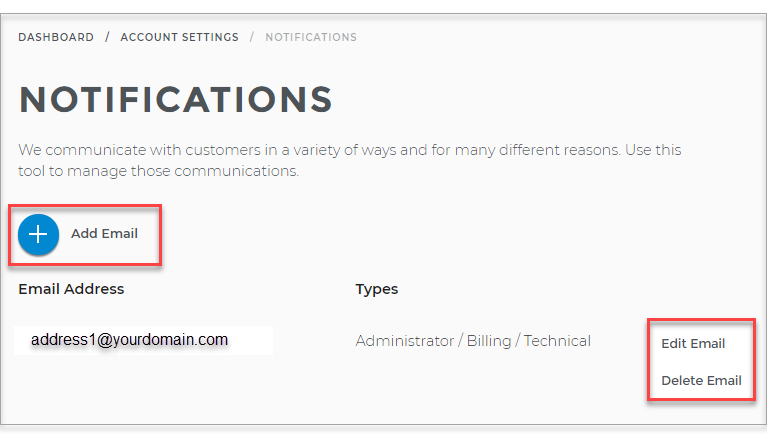Screenshot of a website's notification settings page. The page features a light gray-white background with varying shades of black and gray text. In the top left corner, breadcrumb navigation reads: "Dashboard / Account Settings / Notifications," with "Notifications" grayed out, indicating the current page.

Below the navigation, the title "NOTIFICATIONS" is displayed prominently in all capital letters. A brief description follows: "We communicate with customers in a variety of ways and for many different reasons. Use this tool to manage those communications."

Beneath the description is a red rectangular button. It contains a blue circle with a white plus sign inside and the label "add email" in blackish gray text next to it.

Further down, the page features a section labeled "Email Address" with an input field pre-filled with a placeholder text: "address1@yourdomain.com". To the right of this field is a label that says "Types".

Listed below are the types of email notifications: "Administrator / Billing / Technical".

In the bottom right corner of the page, another red rectangular button allows users to "Edit Email" or "Delete Email."

The colored elements, such as the red rectangles and blue circle, provide contrast against the monochromatic theme of the text.